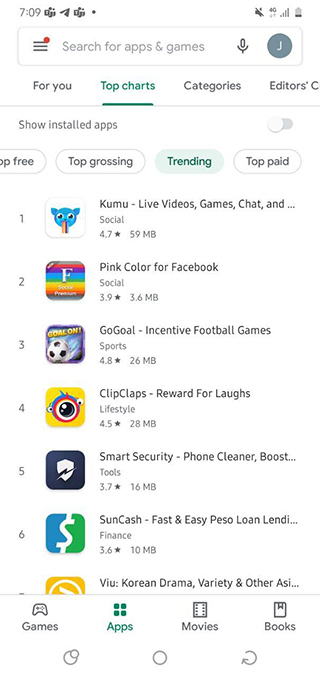At 7 o'clock, the image displays a status bar featuring several icons: a muted speaker symbol, a 4G symbol, a Wi-Fi signal with four bars, and a battery icon indicating low battery. Below this, three vertical bars with a red dot to the right prompt a "Search for apps and games" field, flanked by a microphone icon and a white "J" in the middle of a gray circle.

The next row has several tabs: "For you," "Top charts" (highlighted in green and underlined), "Category," and "Editor's Choice." Below this, a toggle option labeled "Show installed apps" appears, which is switched off. Subsequently, various categories are listed: "Free," "Top grossing," "Trending" (highlighted in green), and "Top paid."

Following this, there is a list of six apps, each accompanied by an icon and description:
1. **Kumu** - Live videos, games, chat.
2. **Facebook** - Displayed with a pink color scheme.
3. **Go Gold Dash** - Incentive football games.
4. **Clip Claps** - Rewards for laughs.
5. **Smart Security** - Phone cleaner and booster.
6. **Sun Cash** - Fast and easy PSO loans.

The list is concluded with an ellipsis, indicating more options are available.